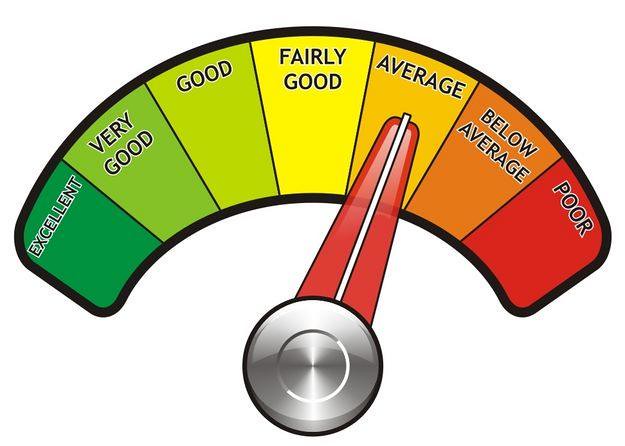The image displays a computer-generated gauge with a half-moon shape and a black outline, resembling a meter or dial reader. The gauge is segmented into seven color-coded sections. Starting from the left, the segments read: "Excellent" in dark green, "Very Good" in a lighter green, "Good" in lime green, "Fairly Good" in yellow, "Average" in light orange, "Below Average" in dark orange, and "Poor" in red. Each label is written in black. The gauge has a red pointer with a silver base and a white stripe, currently indicating "Average."